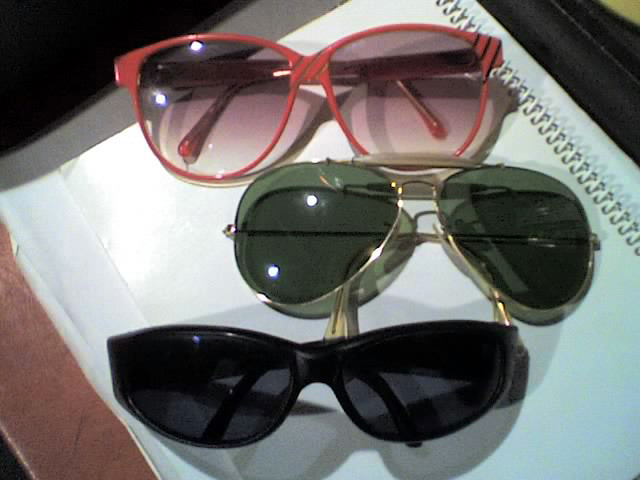This is a detailed photograph featuring three pairs of sunglasses arranged on a white spiral notebook, which itself rests on a brown wooden tabletop. The notebook occupies most of the image, with its spiral binding visible in the upper right corner. A subtle reflection of the spiral is also noticeable. The sunglasses are aligned vertically from bottom to top.

- The bottom pair has a plastic black frame with dark gray lenses, more elongated in shape.
- The middle pair features a golden metal frame, reminiscent of aviator style, with medium-gray lenses. Part of the ear support is visible and distinct.
- The topmost pair has a stylish plastic maroon frame adorned with black striping in the upper right corner and rose-colored lenses. This pair appears rounder in shape. 

Each pair of sunglasses adds a layer of detail and variation to the composition, creating a visually engaging scene.